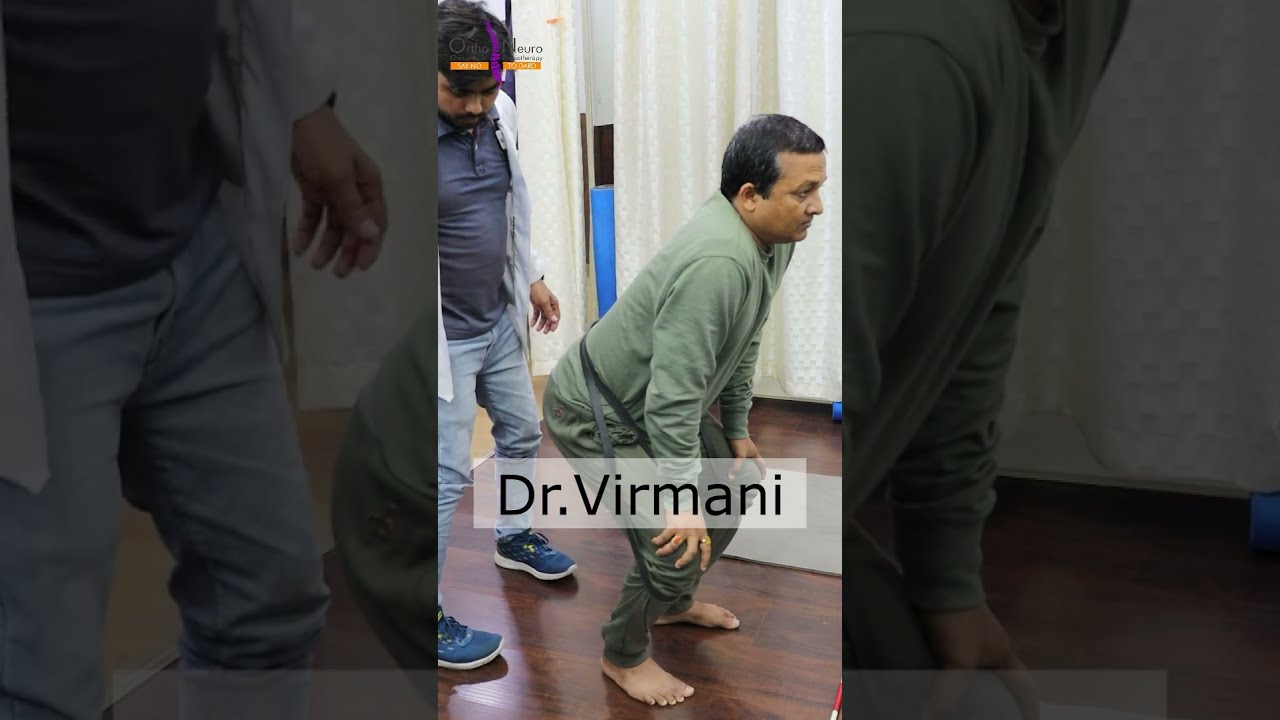In this unusual image, a man is squatting on a dark hardwood floor, barefoot and dressed in a matching olive-green jogging suit. His knees are bent and his hands rest on them. A black bungee cord is wrapped around his waist, extending to his knees. Behind him stands a doctor, identifiable by his white lab coat, blue polo shirt, jeans, and blue tennis shoes. The doctor, who appears to be examining the patient, has "Dr. Vermani" written on his coat. Both individuals have dark hair and seem to be of Indian descent. The setting includes a cream or off-white curtain, likely part of a partition in a patient examination area for privacy.